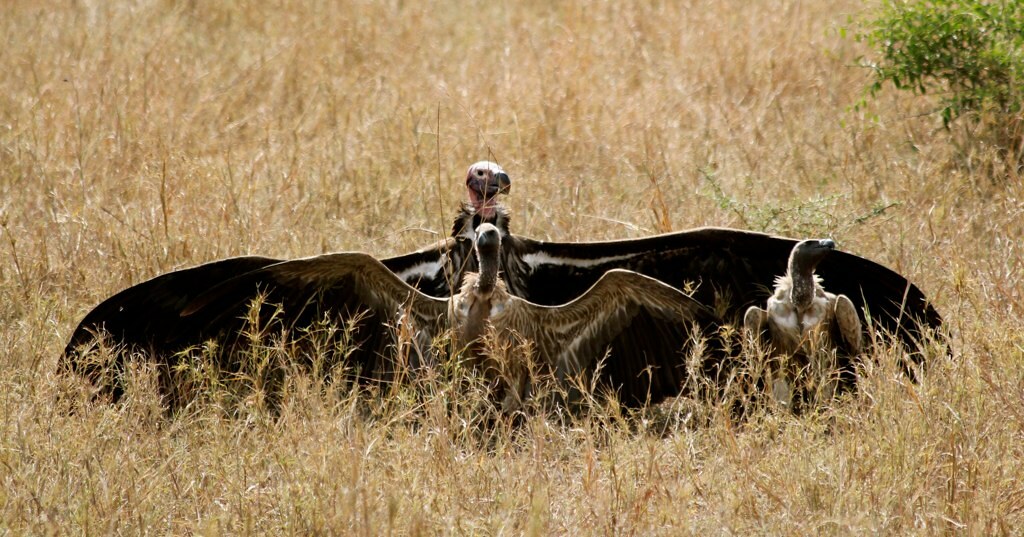The image depicts an outdoor scene on a sunny day, set in a vast field of tall, brown, tan, and yellow grass or wheat. In the center of the image, three birds are prominently featured, likely a falcon or a vulture and its two smaller counterparts, which could be juveniles. The largest bird, with an impressive wingspan, appears to have its wings fully spread. Nearby, one of the smaller birds also has its wings out, while the remaining bird is sitting and looking to the side. In the upper right corner of the image, there is a noticeable green bush, adding a touch of contrasting color to the naturally brown-toned environment. There is no text present in the image. The setting suggests a natural habitat, possibly a farm, in the middle of the day.